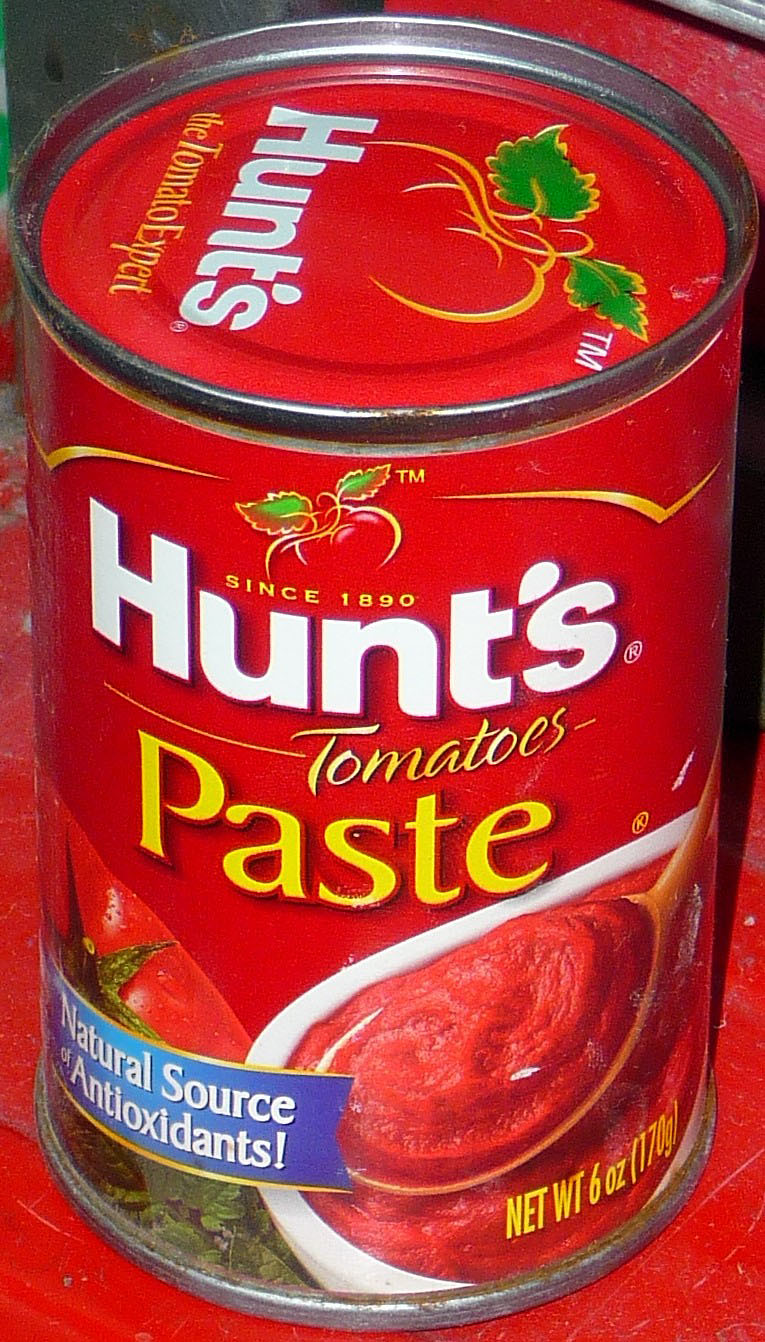This photograph captures a small can of Hunt's tomato paste prominently displayed on a textured, red, cardboard-like surface. The can, primarily deep red with a silver rim, features detailed branding and imagery. On the front label, the text "Hunt's" is written in bold white letters with an apostrophe 'S'. Above this, in yellow, it states "Since 1890" accompanied by an artistic drawing of a tomato with green leaves and a yellow outline. Below, "Tomato Paste" is written with "Tomato" in a lighter yellow and "Paste" in a deeper yellow. A dark blue, v-edged rectangular banner near the bottom-left corner declares "Natural Source of Antioxidants!" in white. The banner partially overlays a detailed image depicting a fresh, deep red tomato paste scooped onto a yellow spoon from a white bowl, surrounded by leafy greens. The can’s top surface continues the branding with "Hunt's" in white and another illustration of a tomato with green leaves. Additionally, the front label notes the net weight of the tomato paste as 6 ounces (170 grams).